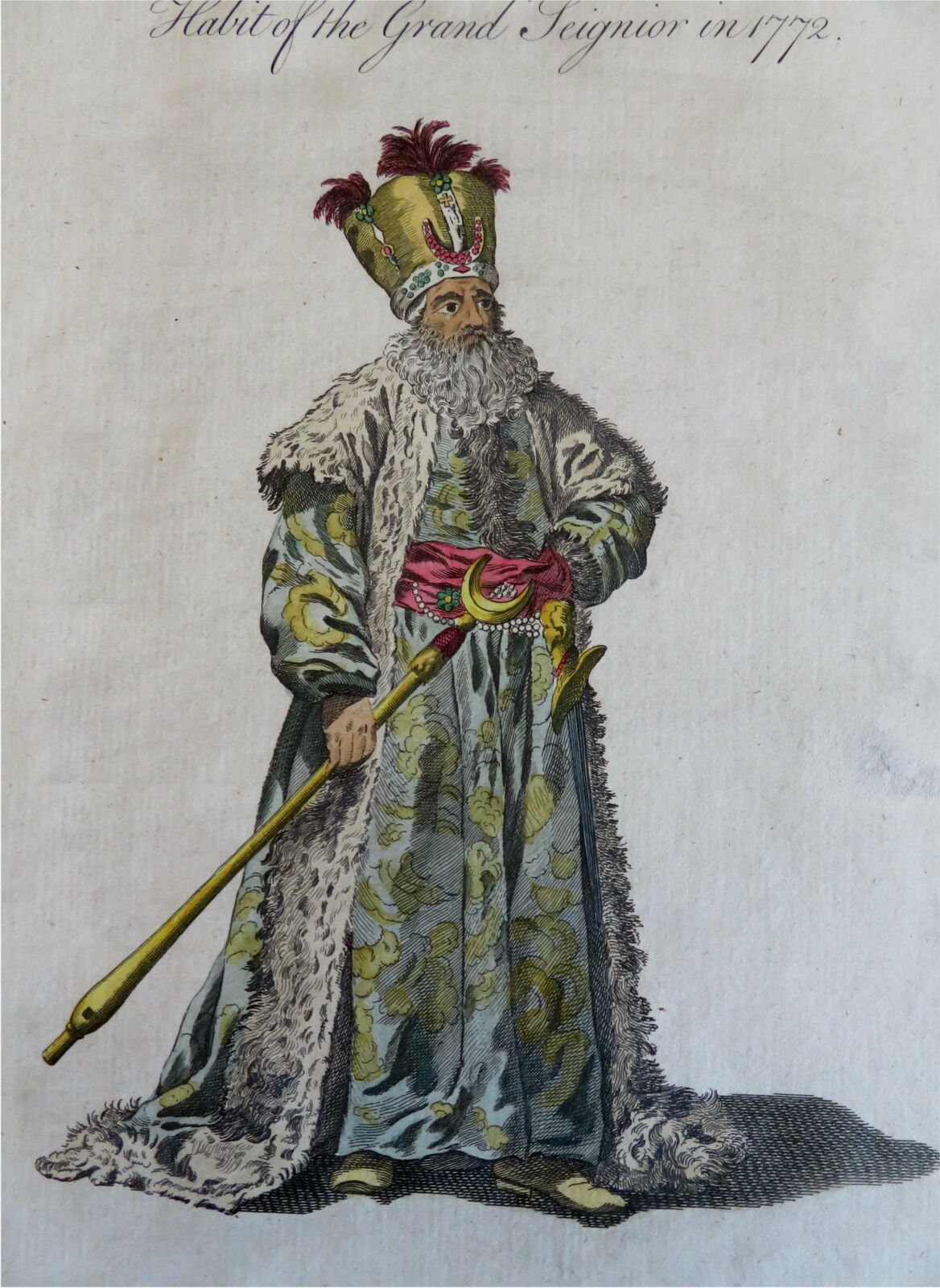This detailed illustration, formatted in portrait mode against an antiqued, fabric-like off-white background, captures an elderly yet dignified man dressed in elaborate regalia. The top of the illustration features the inscription "Habit of the Grand Seigneur in 1772" in an old-style script reminiscent of 18th or 19th-century calligraphy. 

The centerpiece of the illustration is a stately man with a full, somewhat curly white beard. He is holding a gold scepter adorned with a crescent moon motif. Upon his head, he wears a tall fabric crown in gold, accented with a white trim along its base and up the center, and topped with three dark red feather plumes. Below the feathers, a crescent moon motif set with rubies decorates the front of the hat. 

The man is attired in a light blue garment with expansive sleeves, featuring a green floral pattern, worn under a wide, dark red silk belt or sash, which is decorated with pearls and draped flowers. Over this, he dons a luxurious fur stole or shrug, which cascades from his front shoulders down to the floor. His footwear consists of soft, light brown leather boots or shoes. 

The man gazes upward and to his left, presenting a solemn and somewhat stern expression. Overall, his attire and bearing suggest a grand, regal presence, as befitting the title "Grand Seigneur."